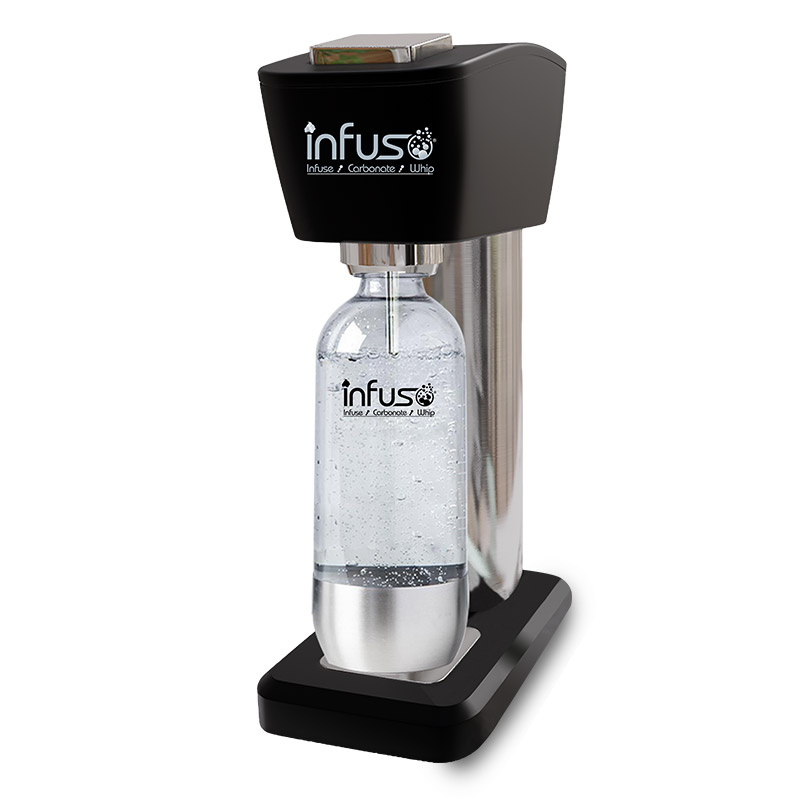The black-and-white photograph, likely an advertisement, showcases a sleek machine designed to carbonate water, known as "infuse" (stylized in all lowercase). The machine features a tapered black top and a black rectangular base, with a silver cylindrical section in between. A clear transparent bottle, positioned under the machine, contains a clear liquid and is connected to a nozzle with a small infuser probe. Prominent white lettering on the front of the machine displays the name "infuse". The bottle also bears the same branding, along with the words "carbonate" and "whip". The image is set against a plain white background, with bright lighting highlighting the details of the product clearly.